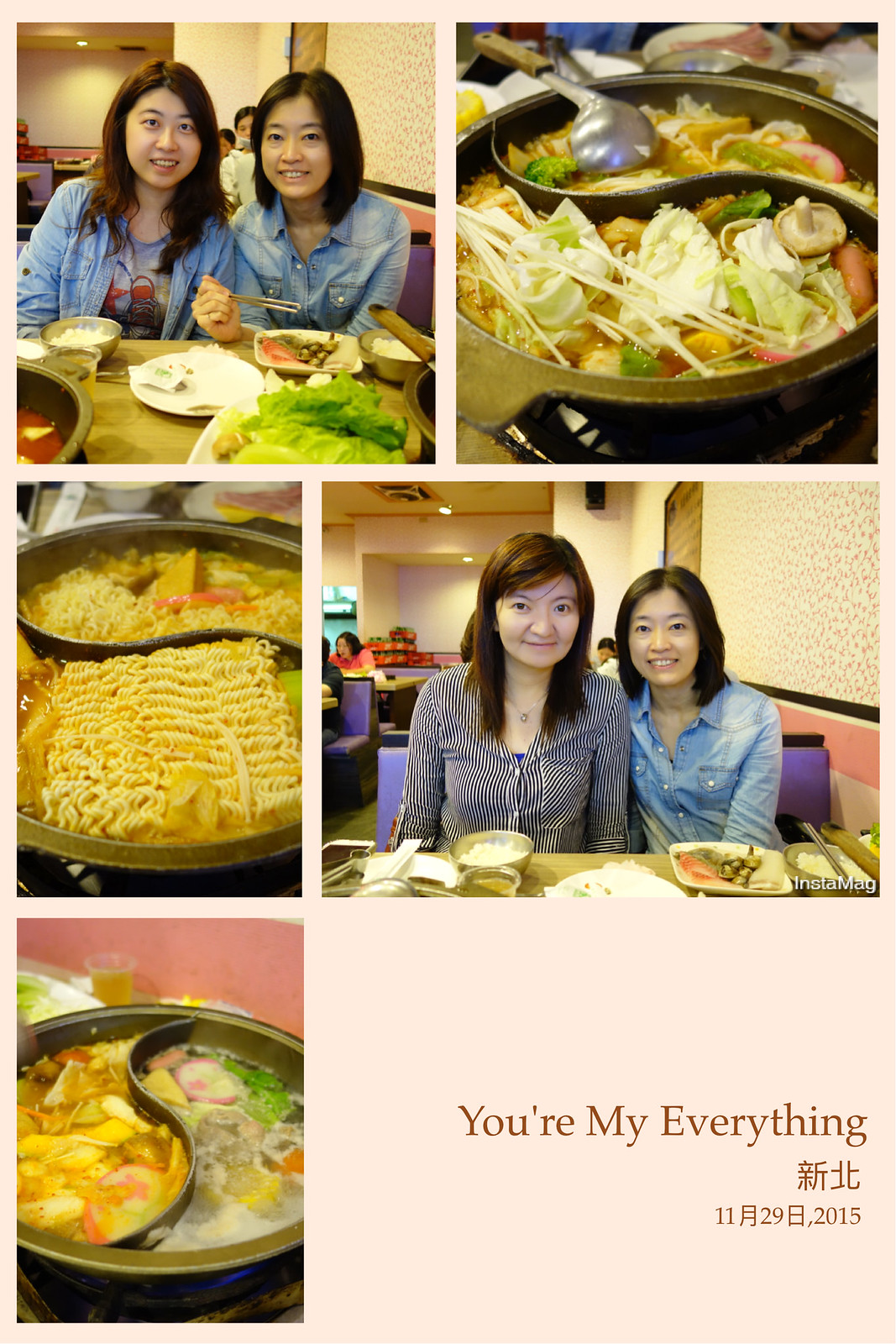The photograph is a collage set against a peach-colored background, featuring five smaller images and a text caption. At the top left, there is a photo of two Asian women seated at a table, both dressed in denim button-up shirts. They are sharing a meal with various dishes spread out before them, including a bowl of rice and some lettuce. One of the women holds chopsticks in her hand. Both are smiling and have dark hair, with one having long hair and the other short.

The top right image is a close-up of a steaming bowl of Asian vegetable soup, featuring visible ingredients like cabbage, carrots, and mushrooms, with a ladle resting on the edge of the bowl. 

In the middle row, the left photo shows a bowl of uncooked ramen noodles sitting prominently in a soup dish. The right photo features two Asian women, one with long brown hair wearing a vertical striped black and white shirt, and the other in the familiar denim shirt with shoulder-length brown hair from the earlier image. They are seated at a booth in a restaurant with food on the table in front of them.

The bottom left image is another picture of a soup bowl, showcasing a different type of Asian vegetable soup. 

Finally, on the lower right side of the collage is the caption text reading "You're my everything," followed by some Asian characters and the date "11-29-2015."